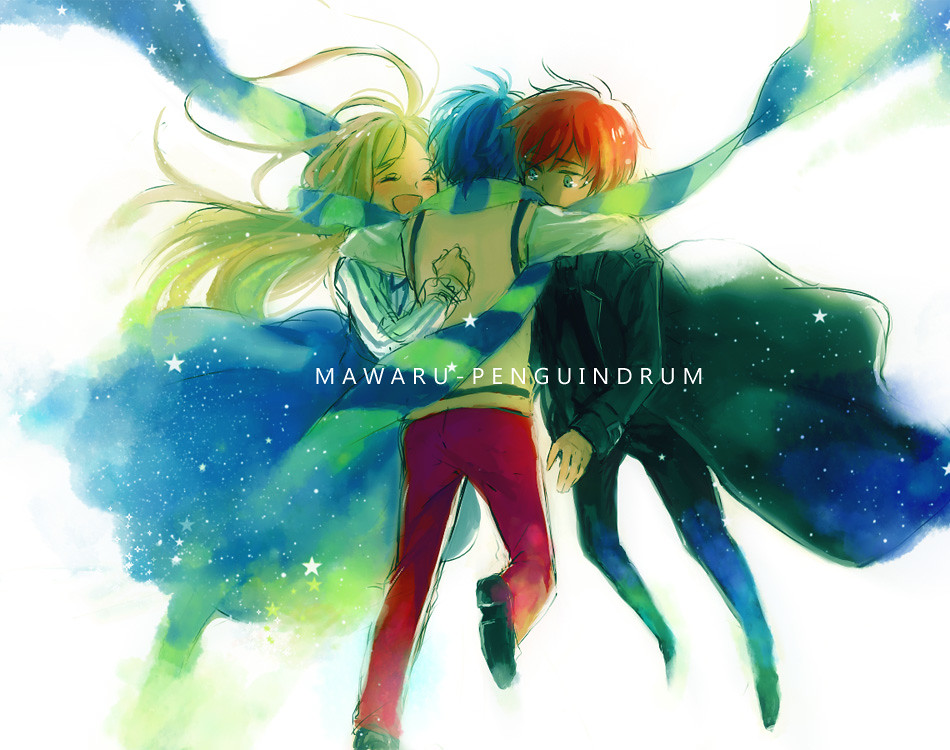The image is a vibrant, anime-style illustration featuring three characters embracing against a white background. At the center is a boy with blue hair, facing away from the viewer. He is wearing a combination of red pants and a striking blue-and-yellow scarf that dramatically swirls around him and the two individuals he is hugging. The scarf extends to various parts of the image, creating a dynamic and whimsical effect.

To the right of the central figure is a girl characterized by her long blonde hair and cosmic blue skirt. She appears to be smiling warmly. On the left stands another boy, identifiable by his reddish-orange hair and dark attire, consisting of a black coat and pants, complemented by a tie. His expression shows emotion, with visible white dots in his eyes hinting at possibly being moved or teary-eyed.

The ensemble creates a mystical, otherworldly atmosphere, capturing a tender moment of connection between the characters, seemingly floating in space. Across the middle of the image, the words "Mawaru Penguin Trump" are inscribed, adding a narrative context to the scene.